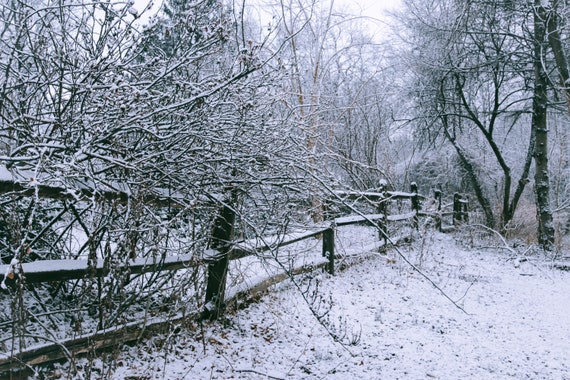The image showcases a sprawling, old, split-rail wooden fence extending from the bottom left corner to beyond the right edge, giving a sense of endlessness. The fence, comprised of three horizontal wooden rails, appears aged and somewhat dilapidated, with sections falling apart. Snow covers the entire scene, blanketing the ground, the fence, and the trees, suggesting a recent light snowfall. To the left of the fence, there are bushes and clumps of grass sporadically protruding through the snow, with some branches leaning down possibly due to the weight of the snow and ice. The barren, blackened trees, some extending beyond the top of the image, dominate the foreground and background, creating a stark contrast against the thick gray sky. The distance is filled with a snow-covered forest and smaller trees, contributing to the desolate, wintry atmosphere. The overall scene conveys a quiet, cold, and untouched winter landscape, frozen in time.